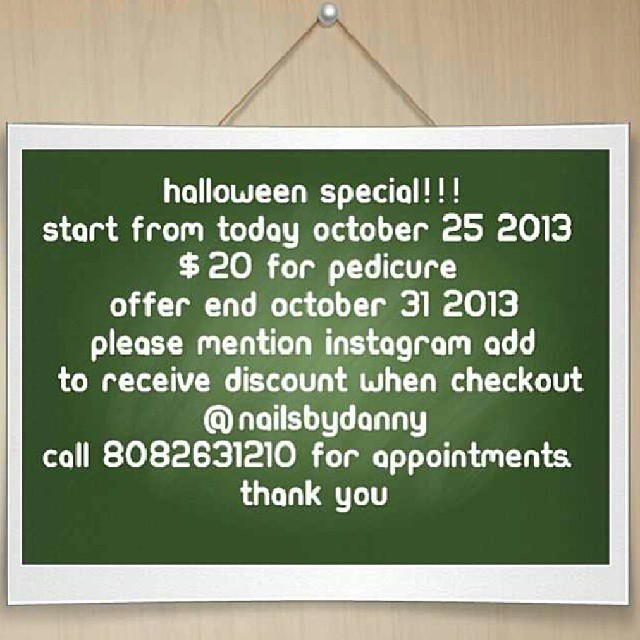The photo showcases a green sign with a silver frame, hanging on a light brown, paneled wall, affixed by a thumbtack or stick pin with strings forming a pyramid shape. The sign features all lowercase, white text and promotes a special offer for Halloween. It reads: "halloween special!!! start from today, october 25th, 2013. $20 for pedicure. offer end october 31st, 2013. please mention instagram ad to receive discount when checkout. at nails by Danny. Call 808-263-1210 for appointments. thank you." The advertisement has a digital, mock-up appearance, and likely aims to attract customers through social media promotions.